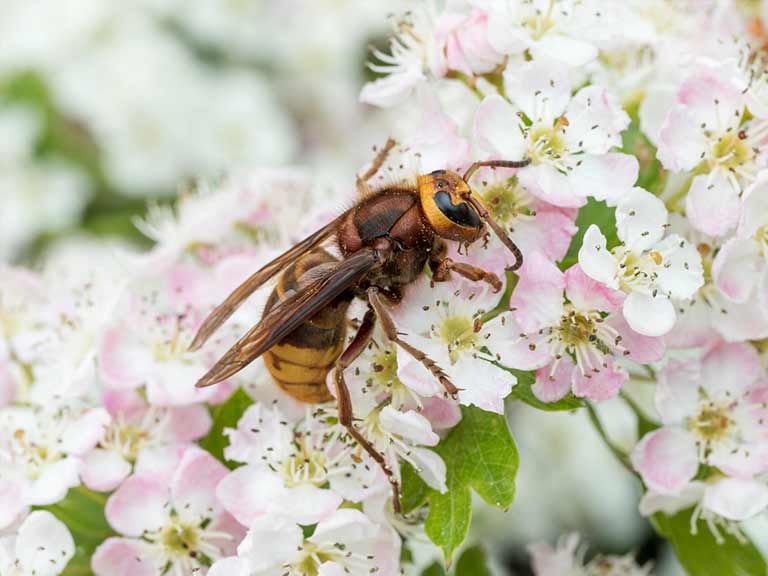In this detailed and vividly clear image, a yellow jacket is prominently featured in the center, engaged in pollinating flowers. The yellow jacket, often mistaken for a bee or wasp, is captured in a slightly tilted position, with its head pointing towards the top right corner and its narrow, brown-tinted wings angled towards the bottom left. Its elliptical black eyes are noticeable on a yellow head with two antennae directed oppositely. The insect's segmented body showcases a striking coloration: a yellow lower back, a predominantly brown upper back, interspersed with segments of dark brown and black.

The yellow jacket is perched on a vibrant cluster of small flowers. These blossoms display a fascinating color palette: some petals are purely white, while others exhibit a combination of pink and white shades, complemented by stamen in the center that are delicate greenish-yellow. The flowers’ elongated stamen adds a striking detail to their appearance. The leaves beneath these flowers are a lush green.

The overall photograph exemplifies the technique of macro photography, focusing sharply on the yellow jacket and the flowers it perches upon while blurring the background. This creates a stark contrast that highlights the intricate details of the yellow jacket and the blooms, epitomizing photographic representational realism. This captivating snapshot, devoid of any textual elements, predominantly features a palette of greens, yellows, browns, whites, blacks, and soft pinks.